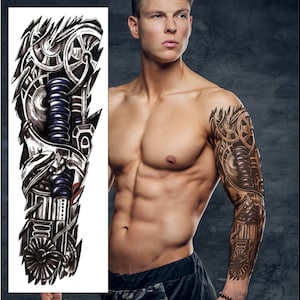The image features a handsome, muscular man posed against a dark background, gazing intensely to the right. He is shirtless, wearing black trunks, with his left arm covered in an intricate sleeve tattoo that spans from his shoulder to his wrist. This detailed tattoo is designed to resemble a robotic arm, featuring intricate mechanical elements like tubes, springs, coils, wheels, and gears in brown rust and silver tones. To the left side of the main image, there is a vertical white rectangle displaying a clearer, more detailed cutout of the tattoo design, emphasizing its cybernetic and mechanical nature.